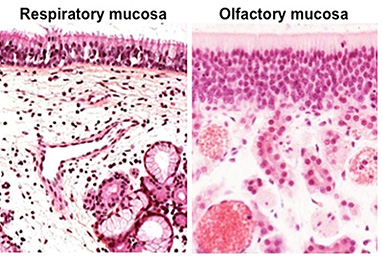This image is a detailed, side-by-side comparison of two microscopic slides, oriented in landscape and divided vertically by a white line. The left slide is labeled "respiratory mucosa" in black letters at the top, and the right slide is labeled "olfactory mucosa," also in black letters. Both slides exhibit cells with varying shades of pink, purple, and red, and feature distinct clusters and distributions of cells.

The respiratory mucosa on the left showcases cells that are more densely packed at the top, gradually dispersing towards the bottom, where larger cells cluster together. Scattered dark-colored specks are visible, denser at the bottom.

The olfactory mucosa on the right, predominantly purplish-reddish in color, starts with a lined arrangement of cells at the top, followed by a tighter cluster of small cells, and finally a more spread-out distribution of larger cells towards the bottom. The slides' resemblance in color and cellular structure, alongside the floating particles in a white background, suggests it is intended for medical training to illustrate mucosal arrangements within the human body.